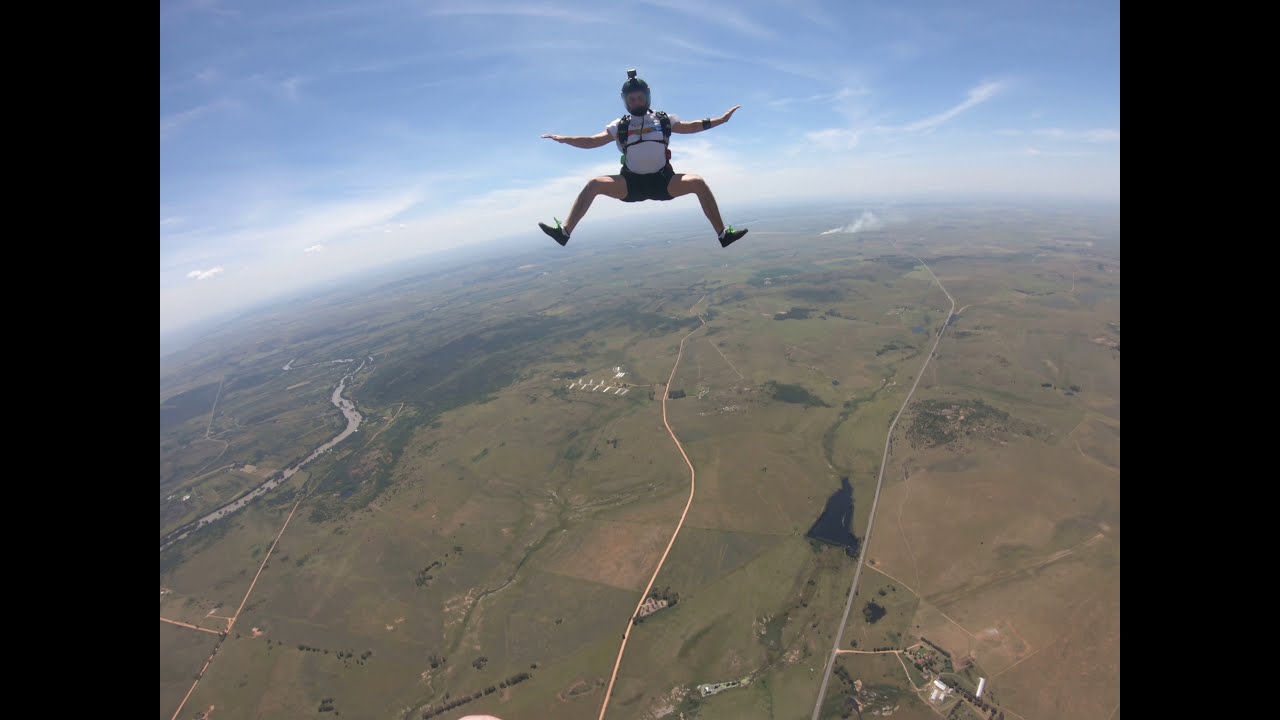This captivating photo captures a skydiver in mid-air, high above the earth. The skydiver wears a helmet mounted with a GoPro camera and is clad in a short-sleeved white shirt, black shorts, and black shoes with green laces. His arms are extended outward while his legs are bent at the knees, giving him a frog-like appearance. The striking backdrop encompasses an expansive bird’s-eye view of the land below, with a distinct curved horizon indicating immense altitude. The landscape beneath is a mix of green and brown hues, interspersed with tiny roads, buildings, and clumps of trees. Notable features include a possible highway or river snaking through the left side of the image, and a patch of white buildings on the bottom right. The sky is a clear blue, adorned with wispy clouds, enhancing the sense of soaring adventure.